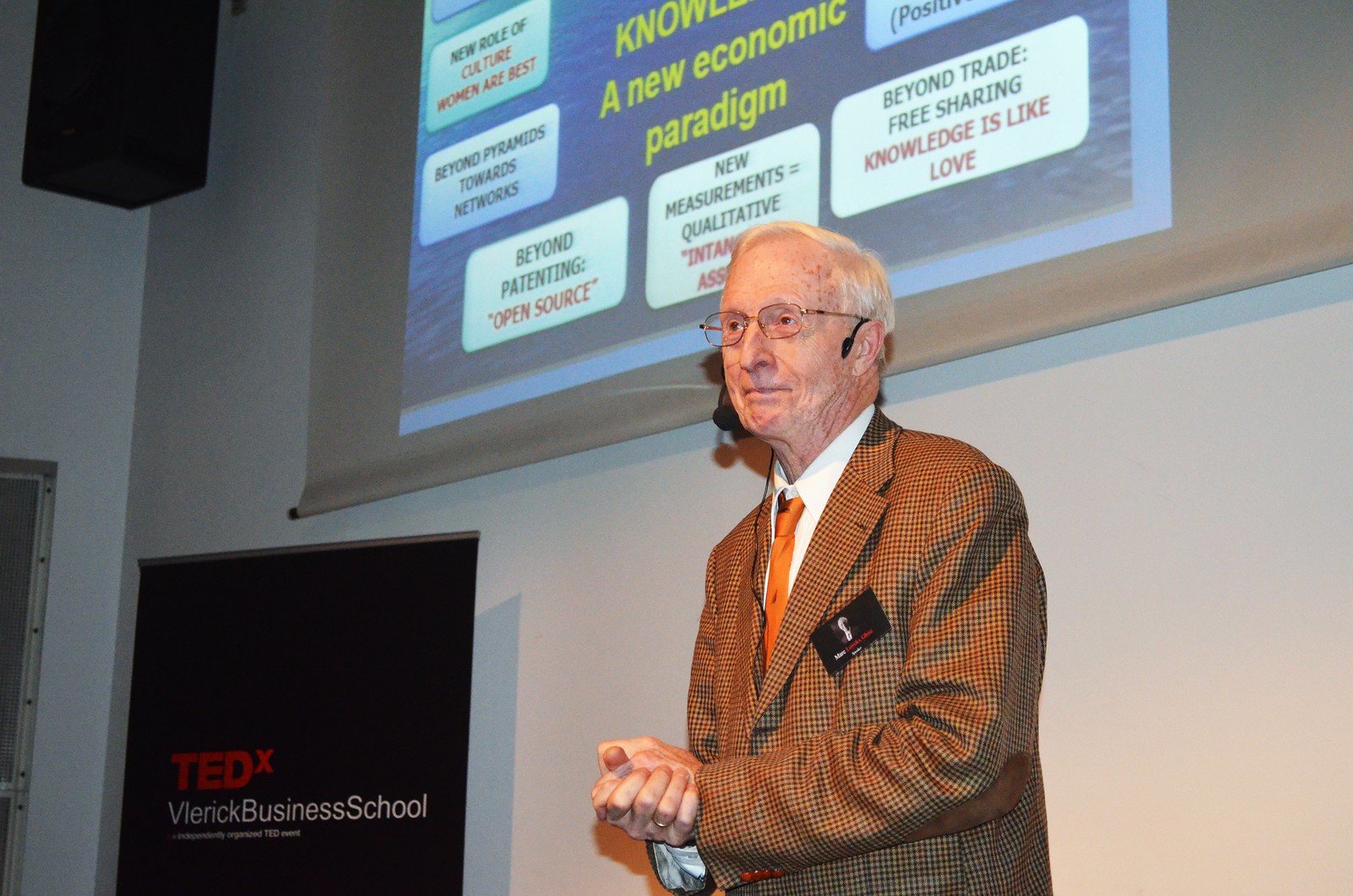The photograph captures an older Caucasian man, likely in his 70s or 80s, with white hair and glasses. He is standing on a stage, possibly having just finished a presentation, as he is holding his hands together, creating the impression of clapping or clasping them. He is wearing a distinctly checkered or plaid suit jacket featuring shades of brown, red, and some orange, paired with a white button-down shirt and a bright orange tie. A small black name tag is visible on his left chest. A headset microphone wraps around his head, placing the mic near his mouth, indicating he has been speaking. The backdrop includes a large screen displaying a slide with numerous white squares filled with texts such as "New Role of Culture, Women are Best," "Beyond Pyramids Toward Networks," "Beyond Patenting, Open Source," "New Measurements, Qualitative," and "Beyond Trade, Free Sharing. Knowledge is Like Love." To his right is a black sign that reads "TEDx Vleric Business School," further emphasizing the formal and professional context of the event. The man appears content, wearing a slight smile, suggesting he is pleased with the proceedings.